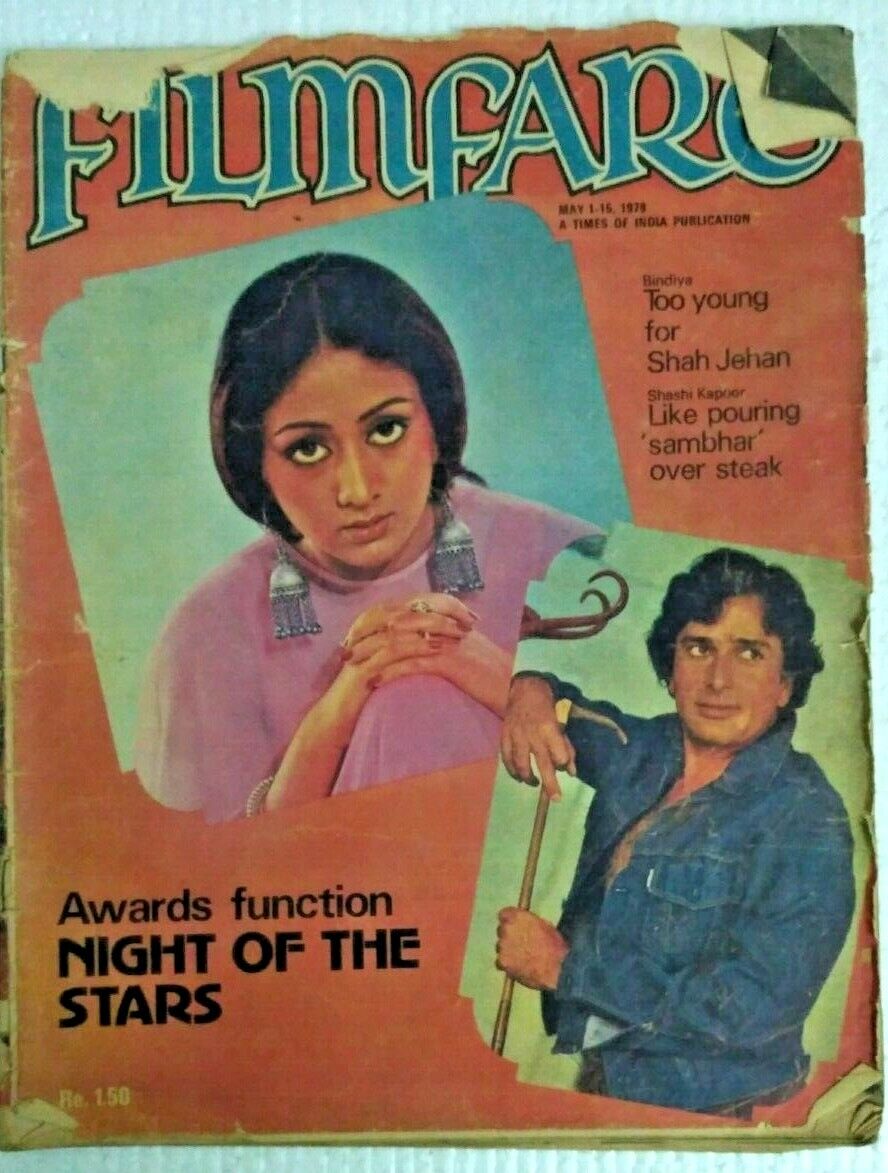This vertical, rectangular image depicts an aged and somewhat deteriorated magazine cover, evident from its frayed edges, slight tears, and the folded upper right corner. The background of the cover is orange-red, adorned with the bold blue title, "Filmfare," in all caps across the top. Due to the damage, portions of the letters, particularly in the upper left and right corners, are obscured. Beneath the title, in smaller black text, is the publication date: "May 1 through 15, 1978," along with the note, "A Times of India publication."

The cover features two prominent photographs. Positioned centrally is a square image of a serious-looking woman with dark hair pulled back. She gazes directly ahead, showcasing long dangling earrings and a pink shirt, with her hands folded neatly in front of her, nails painted. Adjacent to her is a rectangular image of a man clad in a denim jacket, with no visible shirt underneath. His short, curly dark hair frames his face as he looks off to the side, posed with a cane resting on his shoulder.

The lower-left corner of the cover bears the bold black headline, "Awards Function Night of the Stars," emphasizing the magazine's feature. Additionally, the price "R-E-1.50" is noted in the far lower left corner. Despite its damaged state, the magazine vividly captures the essence of its era.